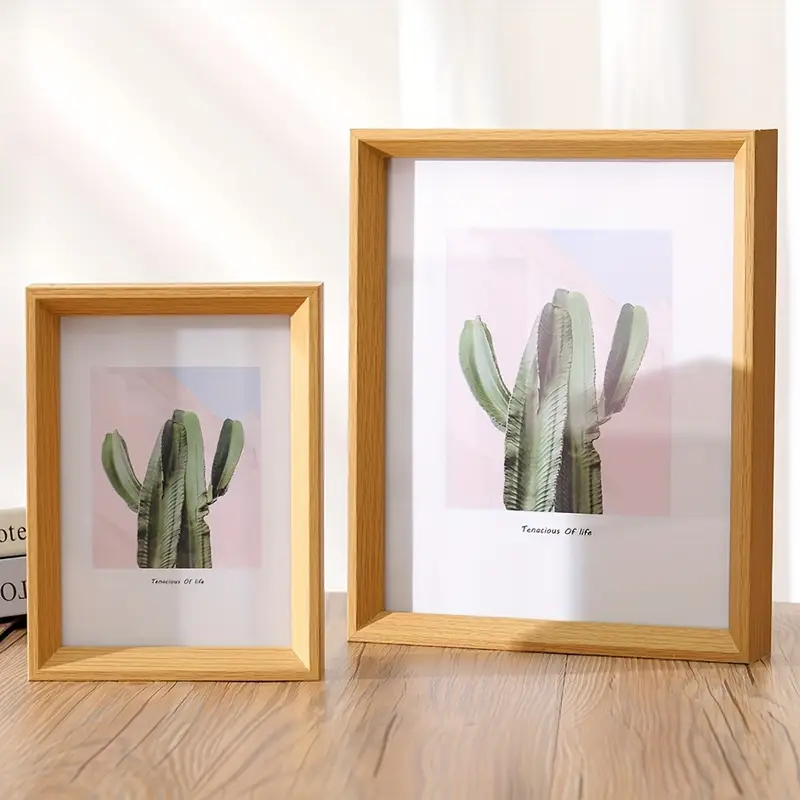The photograph, taken indoors, captures a wooden table with a light brown surface and distinct dark brown vertical striations. The background features a white wall with subtle vertical stripes of light and blue, accented by a blurred white and peach diagonal coloration, possibly created by light coming through a window. On the table, there are two framed art prints. These frames are made of light brown, almost golden-colored wood, and contain identical images depicting a tall, green cactus with horn-like offshoots against a pink and blue sky. Below each cactus image, the text "Tenacious of Life" is printed in black. The frame on the right is notably larger than the one on the left. Additionally, two books are partially visible behind the smaller frame on the left. The overall scene conveys a serene and artistic arrangement.